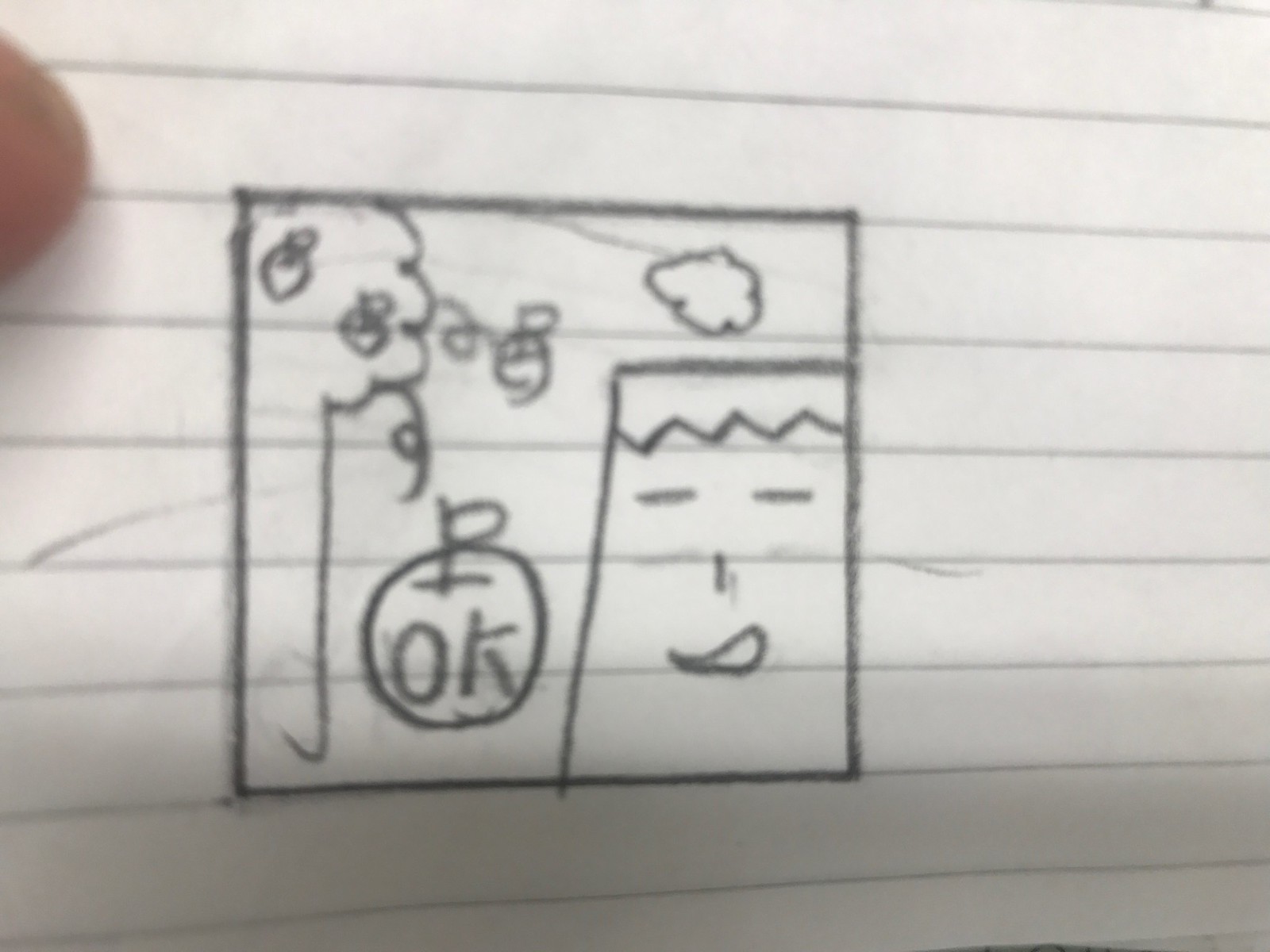The image is a slightly blurry black ink or pencil drawing on white lined notebook paper. The drawing spans approximately five lines in height and is roughly square in shape. On the left side, there's a depiction of a tree with a few circular shapes that resemble apples, inferred from some curly lines suggesting twigs or branches. Below this tree, in the middle of the square, is a larger apple with a stem and a single leaf, inscribed with the word "OK." To the right of the apple is a rectangular, square-headed figure with a simple facial expression, consisting of two horizontal dashed lines for eyes, a vertical line for the nose, and a small semi-circle for a mouth, giving the appearance of a male figure with a smiling expression and a jagged hairline resembling peaks or triangles. Above this figure, there's a fluffy object that looks like a cloud. The paper features black horizontal lines, and there's a hint of a thumb or finger in the upper left corner of the photo.